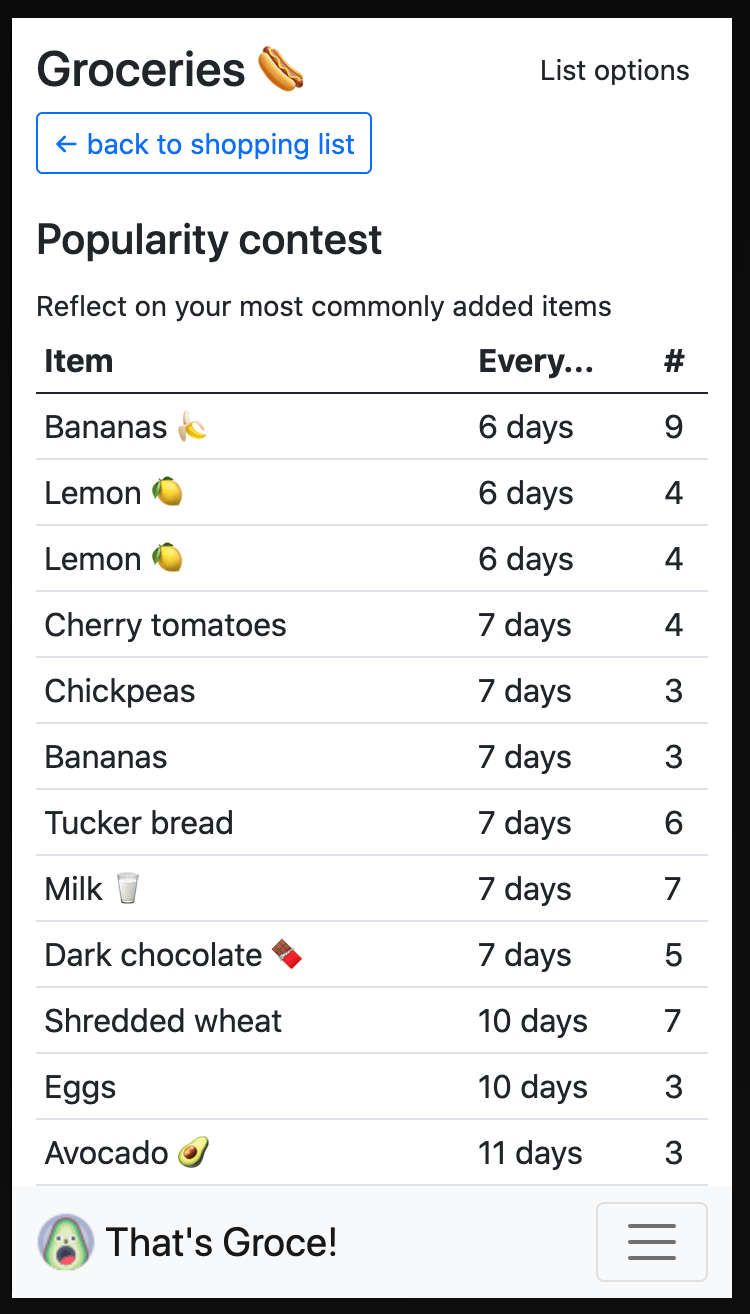Here is a detailed and cleaned-up caption for the image described:

---

The screenshot displays a section from a grocery list application. In the upper left-hand corner, there is a black bar with the word "Groceries" written on it. Adjacent to this text is a hot dog icon, and on the far right, there are options for managing the list. Below the "Groceries" header, there is a white box with a blue border and blue text that reads "Back to shopping list."

Beneath this, the phrase "Popularity contest" is displayed in black font, followed by a prompt to "Reflect on your most commonly added items." 

Next, there is a table-like structure with three columns. The first column is labeled "Item," the second column is marked "Every..." and ends with ellipses (…), and the third column is denoted with a pound sign (#). A line separates the column headers from the list below.

The listed items include:
- Bananas: every 6 days (#9)
- Lemons: every 6 days (#4)
- Lemons (appears again): every 6 days (#4)
- Cherry Tomatoes: every 7 days (#4)
- Chickpeas: every 7 days (#3)
- Bananas (appears again): every 7 days (#3)
- Tucker Bread: every 7 days (#6)
- Milk: every 7 days (#7)
- Dark Chocolate: every 7 days (#5)
- Shredded Wheat: every 10 days (#7)
- Eggs: every 10 days (#3)
- Avocado: every 11 days (#3)

These items are presented against a white background and are written in black font. 

At the bottom of the screen, on the left-hand side, there is a phrase "That's gross!" emphasized with an exclamation point. On the far right, there is a button with an icon of three parallel lines, indicating a menu option.

---

This caption captures all the details from the image, structured clearly and concisely.